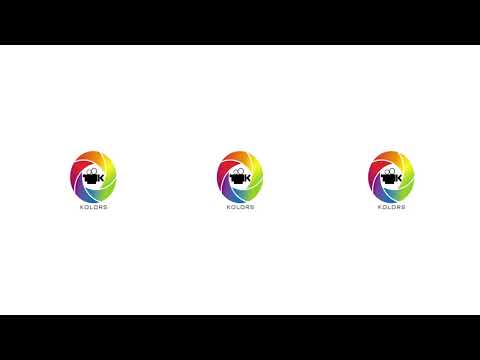The image depicts a simplistic, computer-generated design on a plain white background, presented in landscape orientation. Centered along the midline of the photo are three identical logos, arranged side-by-side horizontally. Each logo features an old-style, black movie camera with two reels on top, pointing to the left. To the right of the camera is the letter "K," and around the camera is a circular rainbow-colored design that spirals with colors transitioning from red on the left through orange, yellow, green, blue, and violet, describable as bent, curved triangles. Beneath each emblem, in light gray block letters, is the word "KOLORS," spelled with a "K." The background of the camera is within a pentagon shape, and the entire vibrant logo suggests an association with technology. The overall composition is tidy, with a repeating pattern that is pleasant in its simplicity.